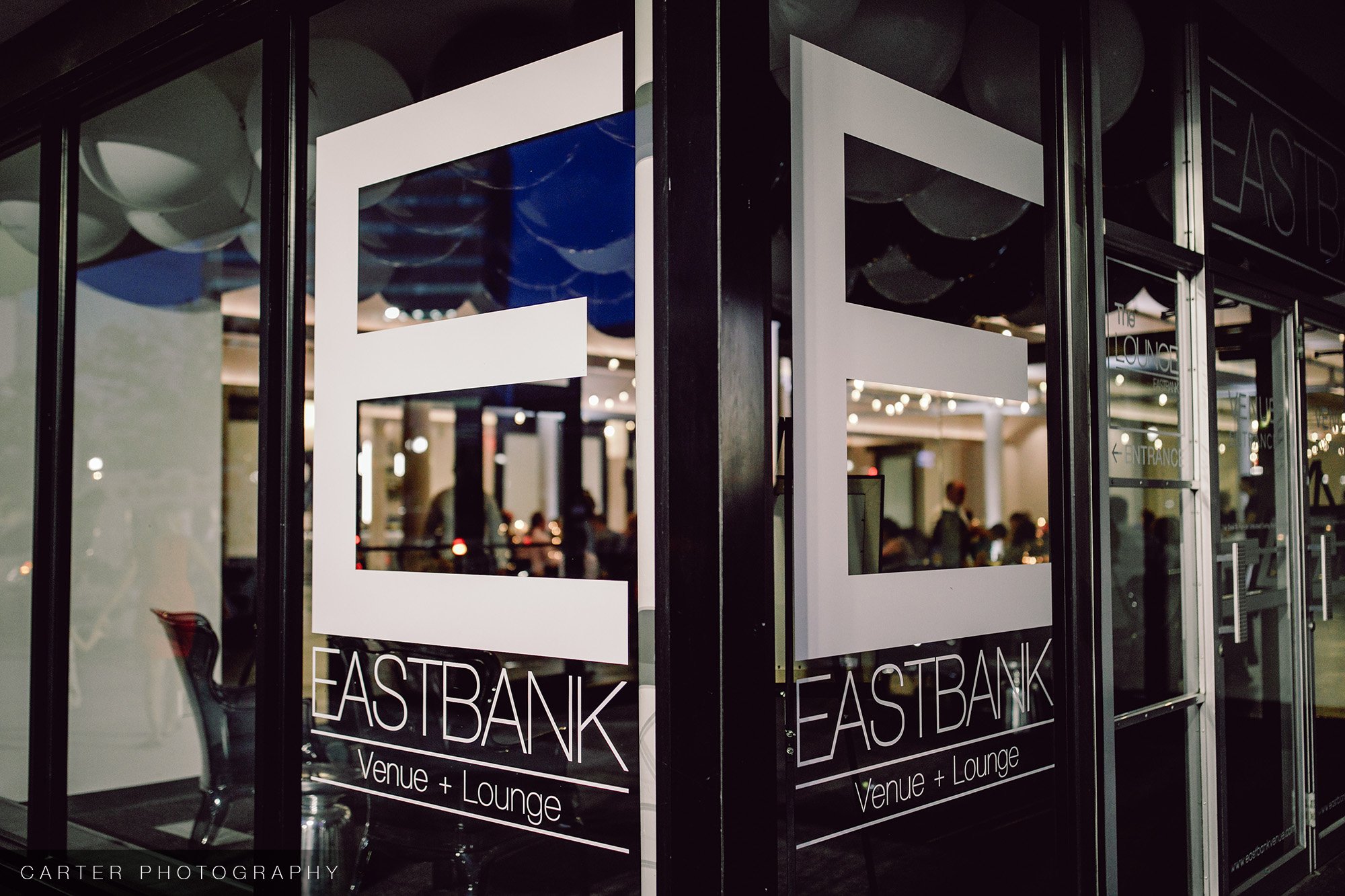This photograph, taken by Carter Photography, captures the exterior of the East Bank venue, a lounge and event space identified by large white capital letter 'E's on two of its front corner windows. Directly beneath the 'E's, the words "East Bank" are displayed, followed by "venue plus lounge" separated by white lines. The storefront features clear glass windows and a double set of silver-framed doors. Visible through the windows are blurred figures, possibly patrons, seated in black chairs surrounded by celebratory balloons, both white and black, hinting at a function inside. The interior is dimly lit with small lights along the ceiling, adding to its festive atmosphere. The lower left corner of the image bears the watermark "Carter Photography."